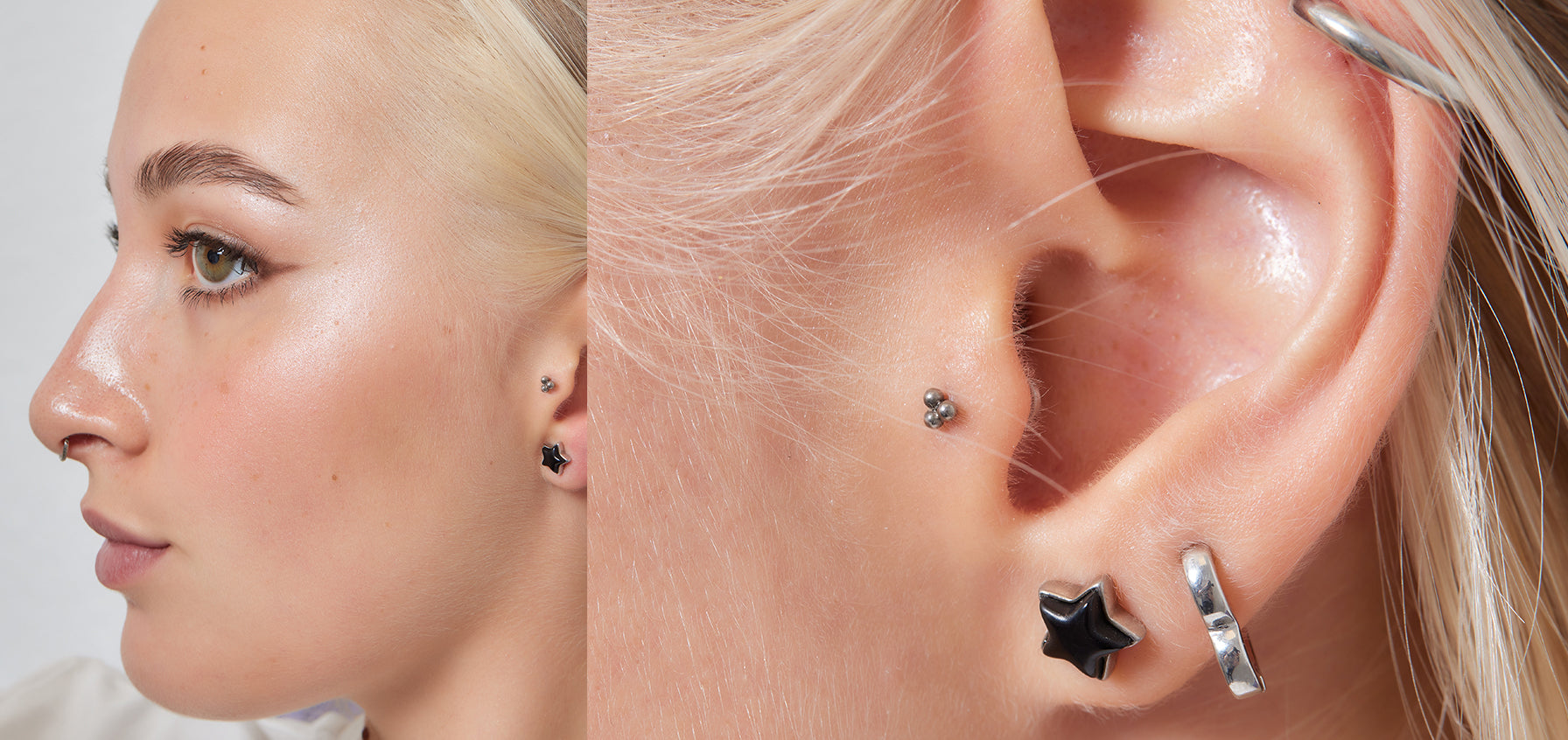The photograph showcases a young blonde woman’s profile combined with a close-up of her ear jewelry, designed for a product page selling earrings. The left third features the woman’s neutral expression, highlighting her nose ring, greyish-brown eyes, and partially visible lips, set against her medium-colored skin tone and cascading blonde hair. The right two-thirds zooms in on her ear, revealing four distinct piercings. The standard piercing contains a black star encased in a silver star-shaped setting. Alongside that, there’s a silver loop piercing, and at the top of her ear, a silver ring encircles her outer cartilage. In the hard cartilage section, the photograph accentuates a detailed piercing featuring three small silver balls. The intricate jewelry design highlights various ear adornments, blending black and silver elements to create a stylish and cohesive look.